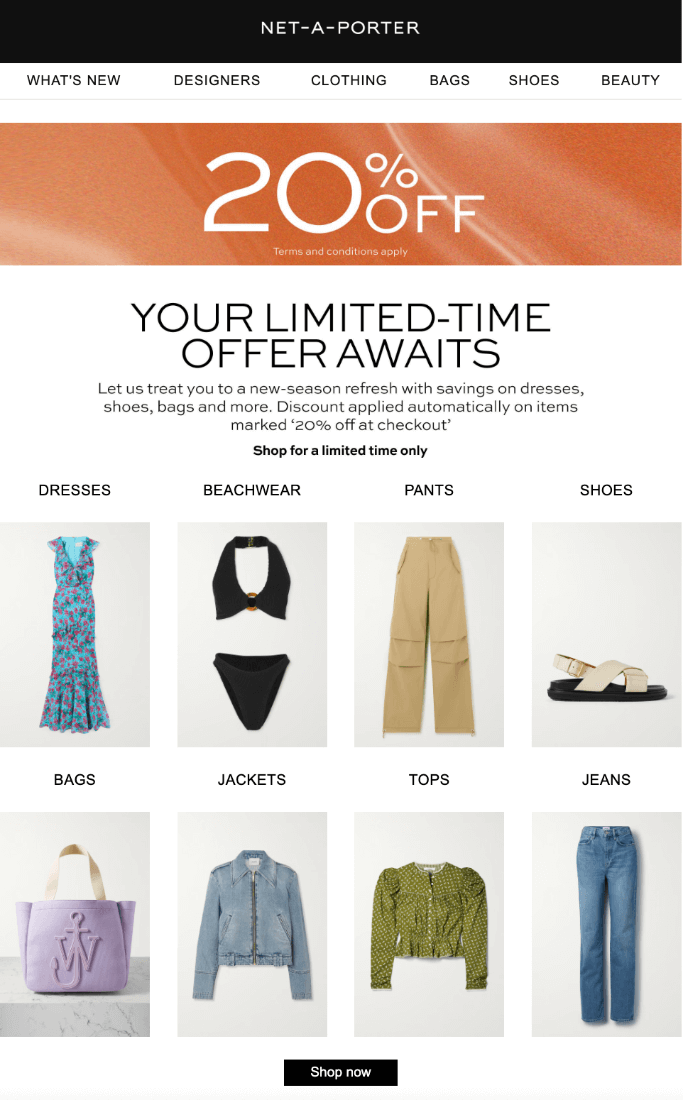The screenshot captures the homepage of the Net-A-Porter web application. At the very top of the page, a bold white "Net-A-Porter" logo is prominently displayed on a sleek black banner. Directly below are navigation tabs: "What's New," "Designers," "Clothing," "Bags," "Shoes," and "Beauty," allowing for easy browsing through various product categories.

A striking orange banner at the top of the page announces a "20% off" promotion in the largest font size on the screen, ensuring it grabs attention immediately. Below in smaller white font, it states, "terms and conditions apply," subtly indicating the fine print.

The background transitions to white, where an inviting message reads, "Your limited time offer awaits. Let us treat you to a new season refresh with savings on dresses, shoes, bags, and more. Accounts applied automatically on items marked 20% off at checkout." This text is designed to persuade customers to take advantage of the sale.

In bold black font, a reminder is issued: "Shop for a limited time only." Beneath that are visually arranged categories including "Dresses," "Beachwear," "Pants," "Shoes," "Bags," "Jackets," "Tops," and "Jeans," each illustrated with a representative item. Under the "Bags" category, there is a standout item: a purple beach tote adorned with an anchor and the letter "W."

At the bottom of the page, a conspicuous black button labeled "Shop Now" beckons users to commence their shopping spree.